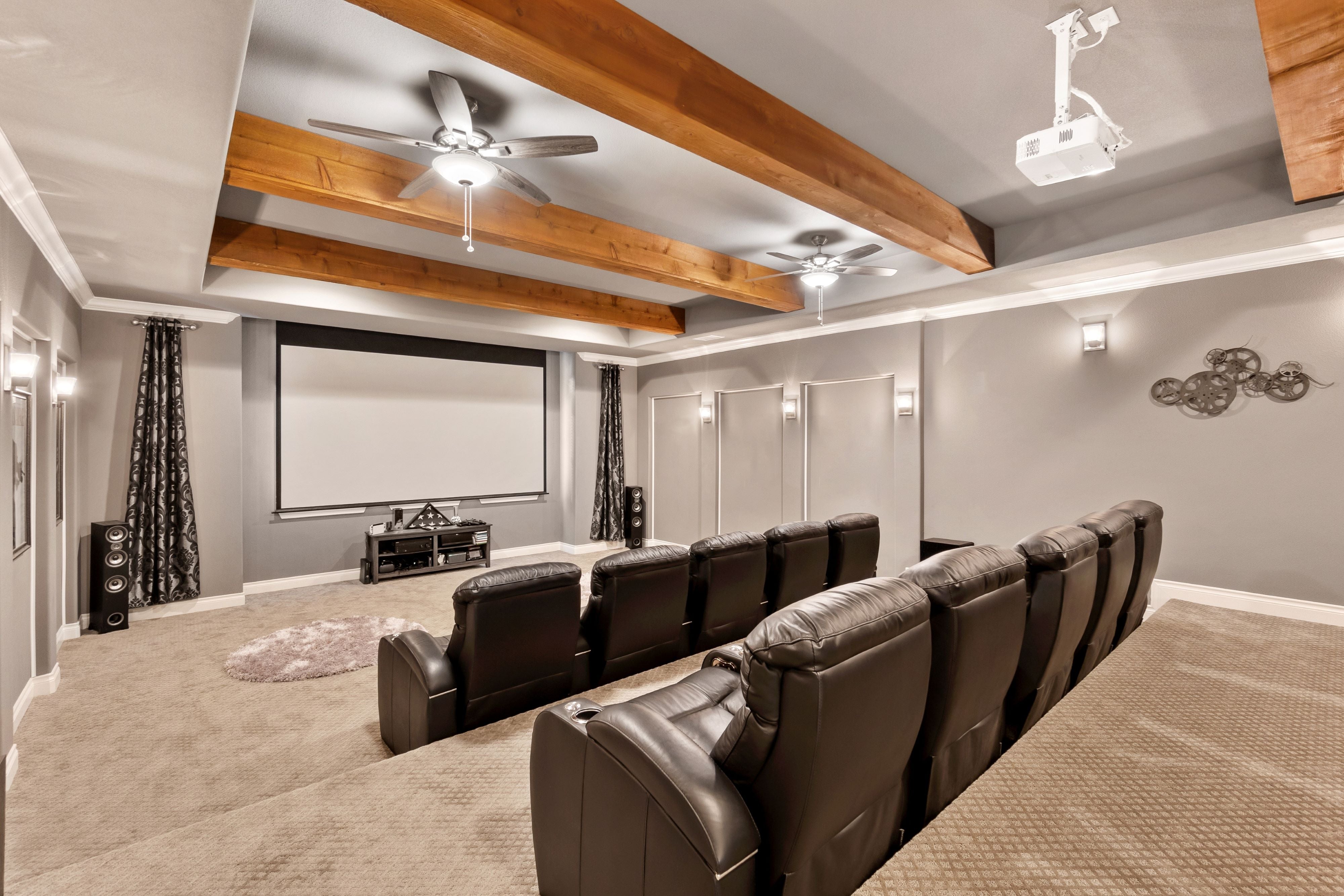The photograph showcases an elaborate home theater room with three distinct, carpeted tiers. The room is designed for an immersive cinematic experience, featuring gray-painted walls accented with oak-colored beams on the ceiling. Overhead, two ceiling fans and a white projector are prominently visible. The centerpiece is a large projection screen at the front of the room, flanked by black and gray curtains and accompanied by black speakers.

The seating consists of two rows of plush, brown leather recliners, with each row accommodating five seats. Situated on different levels, this tiered seating mimics a commercial movie theater setup. On the front-most level, beneath the screen, a table displays a folded American flag, a poignant tribute likely indicating a military connection, surrounded by various items and books.

Decorative elements include sconces lining the walls, a decorative movie reel with four reels, and film-related posters. The flooring features a tan carpet with a gray rug at the front. The room's muted color palette lends a cozy atmosphere, and the presence of rafters and eaves adds to the architectural interest. Additional features such as a media console table and ceiling-mounted fans further enhance the room's functionality and aesthetic.